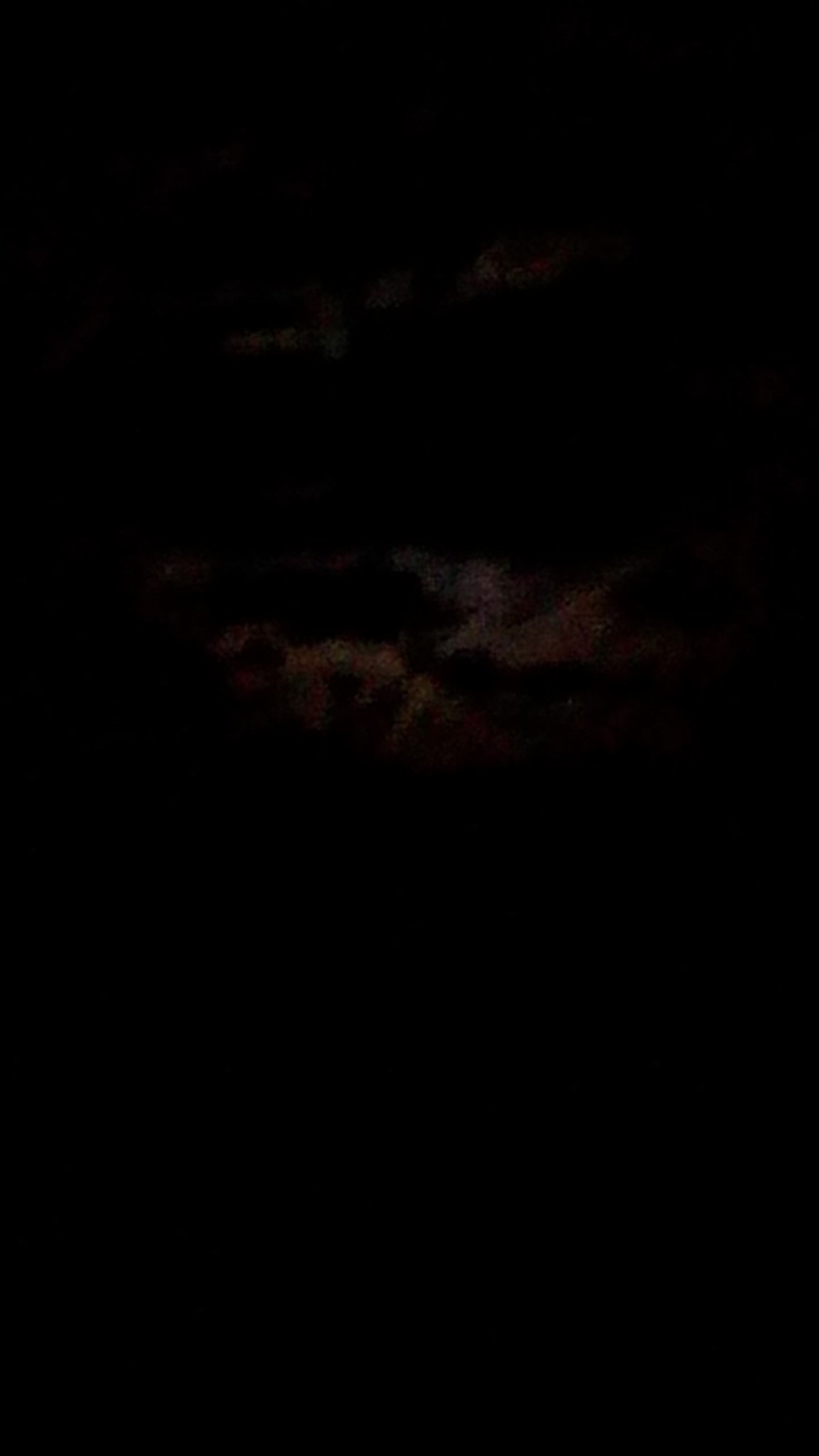The image is predominantly a black rectangle, encompassing approximately 95-98% of the frame. In the center, slightly above the midpoint, there is a faint, indistinct shape. This shape, appearing as a ghostly figure in very dark grey, possibly tinged with dark orange or light brown, vaguely resembles clouds or flowers. Its presence is the sole discernible element in an otherwise nearly pitch-black photograph.